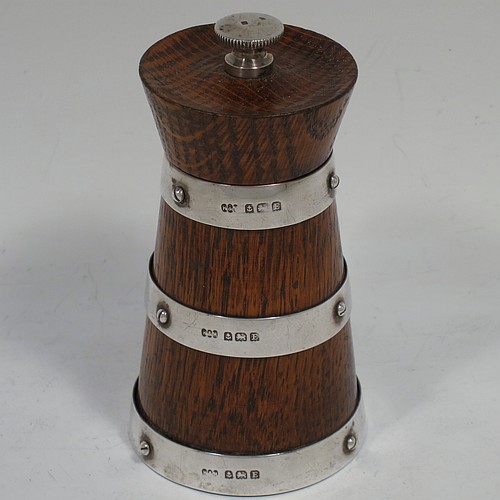This image depicts a dark brown wooden spice grinder, potentially used for either salt or pepper, against a medium gray background. The grinder is cylindrical, with a distinctive hourglass-like shape—starting wide at the bottom, narrowing toward the upper middle, and expanding slightly again near the top. The body of the grinder features three stainless steel bands, each fastened with two visible screws and bearing an illegible stamp or embossing. These metal bands are positioned at the base, the middle, and near the neck where the upper part of the wood meets the lower part. The top of the grinder features a small gear-like adjustment knob, likely designed to regulate the coarseness of the grind. The wood surface exhibits black grain lines, adding to its old-fashioned appearance.